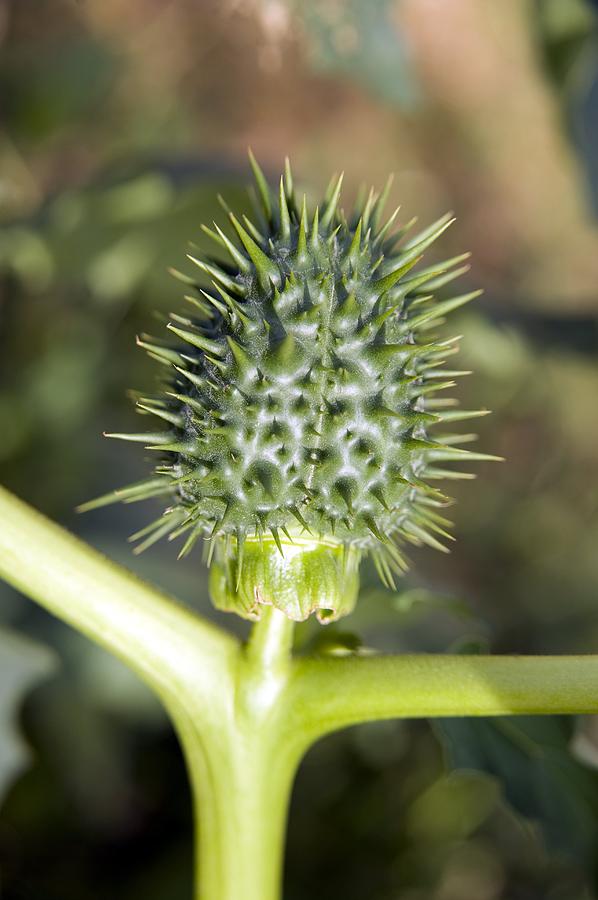The photograph presents an intricately detailed, close-up view of a plant, likely captured using macro photography, with the primary focus on the upper stem and bud. The plant's stem, a light green color, extends from the bottom of the image and splits into multiple directions: left, right, and upwards. Prominently in the center, a spiky, dark green bud is visible, giving the impression of a head adorned with spiky hair. Around the base of the bud, there is a frill-like structure contributing to its distinct look. The blurred background, featuring hues of green, yellow, blue, and a triangular section of orange towards the top-middle, creates an impressionistic effect that highlights the plant's details starkly against a dreamy, soft-focus backdrop. The composed scene evokes the image of a humanoid figure with outstretched arms and a spiky head in a world of vibrant, diffused colors.